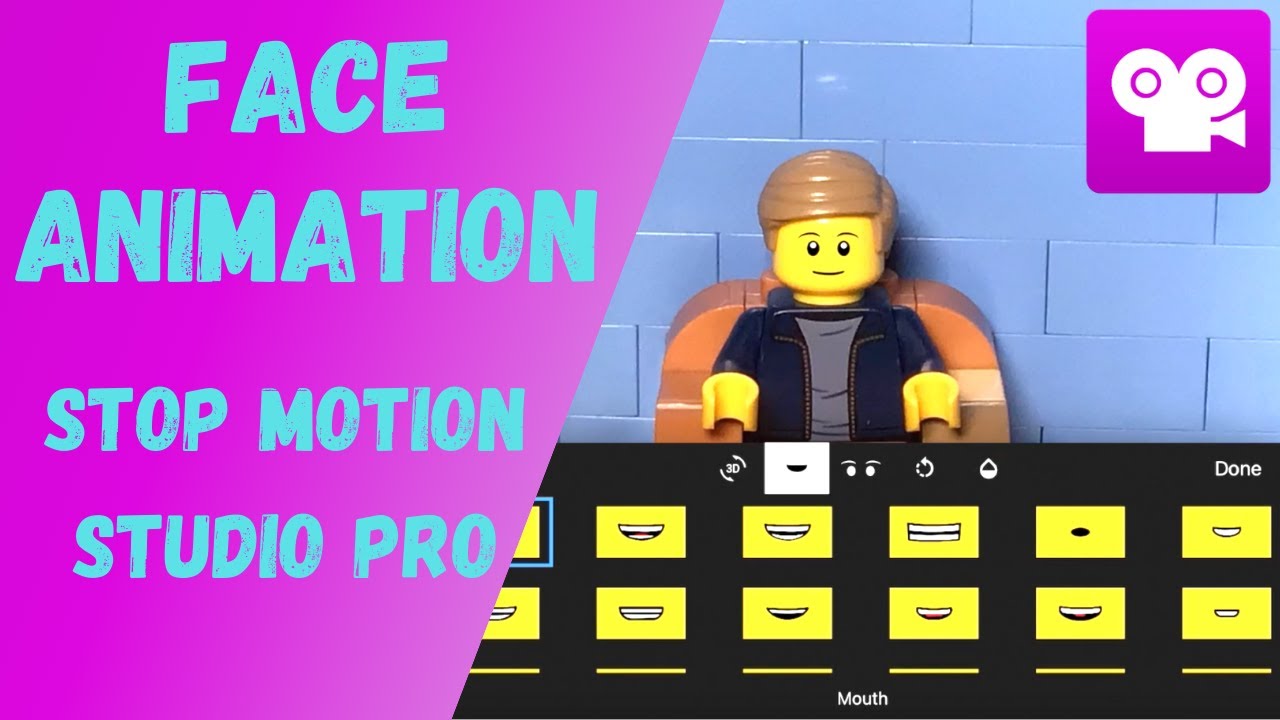The image is a screenshot from a YouTube video, showcasing the Face Animation Stop Motion Studio Pro. The foreground features a prominently displayed Lego man seated on a couch against a gray brick wall, dressed in a black vest with iconic yellow hands and face. The left-hand side of the image presents a text banner in capitalized, teal-colored letters that read "Face Animation Stop Motion Studio Pro" against a pink background; the text has a hand-drawn and solid design mix. The right-hand side displays a white video camera logo with two eye-like circles, set against a pink background. Beneath this logo, various mouth options for the Lego figure are shown, illustrating the software's capability to modify facial expressions in stop-motion animations.